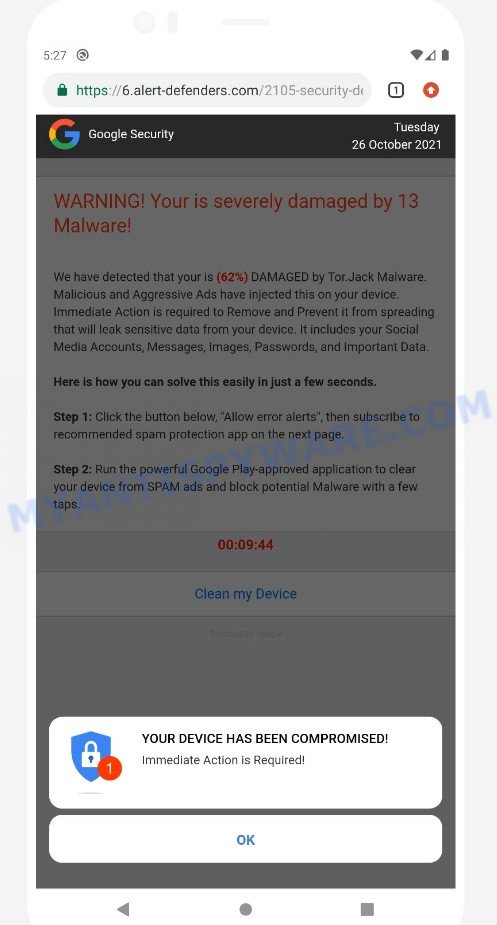The image shows a Google security alert with an opaque gray filter overlay, making the text partially obscured. At the top, there is a URL, followed by a heading reading "Google Security Alert" dated Tuesday, 26th October 2021. The alert warns that "Your device is severely damaged by 13 malware." It specifies that "62% of your device is corrupted by Tor jack malware," and emphasizes that "malicious and aggressive ads" have injected this malware onto the device. The alert urges immediate action to prevent the spread of malware that could leak sensitive data, including social security numbers, social media accounts, messages, images, passwords, and other important information.

The alert provides steps to resolve the issue:
1. Click the button below to allow the error alert and subscribe to the recommended spam protection app on the next page.
2. Run the Google Play-approved application to clear the device of spam ads and block potential malware with just a few taps.